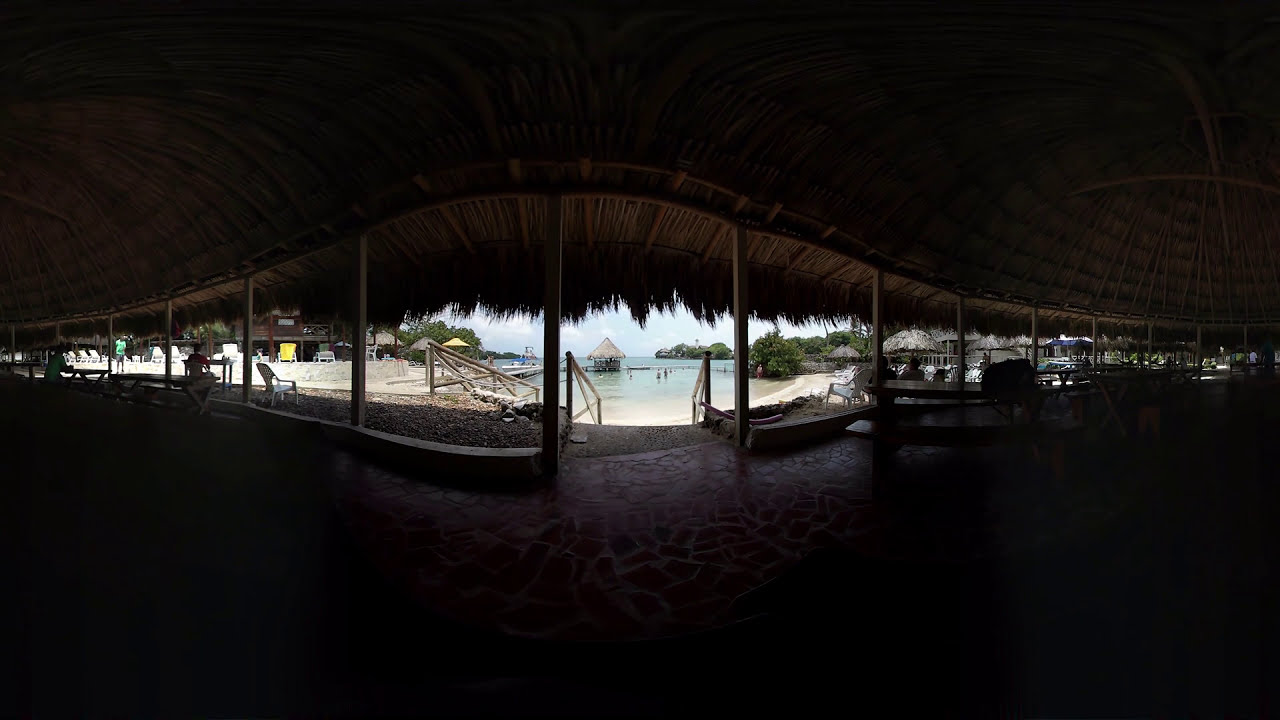This detailed photograph captures a picturesque beach scene as viewed from inside a large, open-air pavilion with a unique thatched roof made of straw or bamboo. The pavilion has a redstone-tiled floor and wooden pillars supporting its grass-like roof which extends slightly beyond the ceiling, providing shaded protection. Inside, there are brown benches between the pillars and various tables scattered around. To the left, a person in a turquoise t-shirt sits, while another person in a red t-shirt is seated nearby. You can spot more individuals on the far right.

The architecture of the pavilion appears skewed due to the photograph's warped perspective, giving it a curved look that might not be natural. This semi-open structure opens up to a wooden staircase leading down to a small beach and a squared-off waterway that likely connects to a vast ocean. The surrounding area is bright with blue water, green trees, and additional small cabanas with similar roofs scattered near the water. The ambiance is tranquil, with people wading into the clear blue water under a clear blue sky.